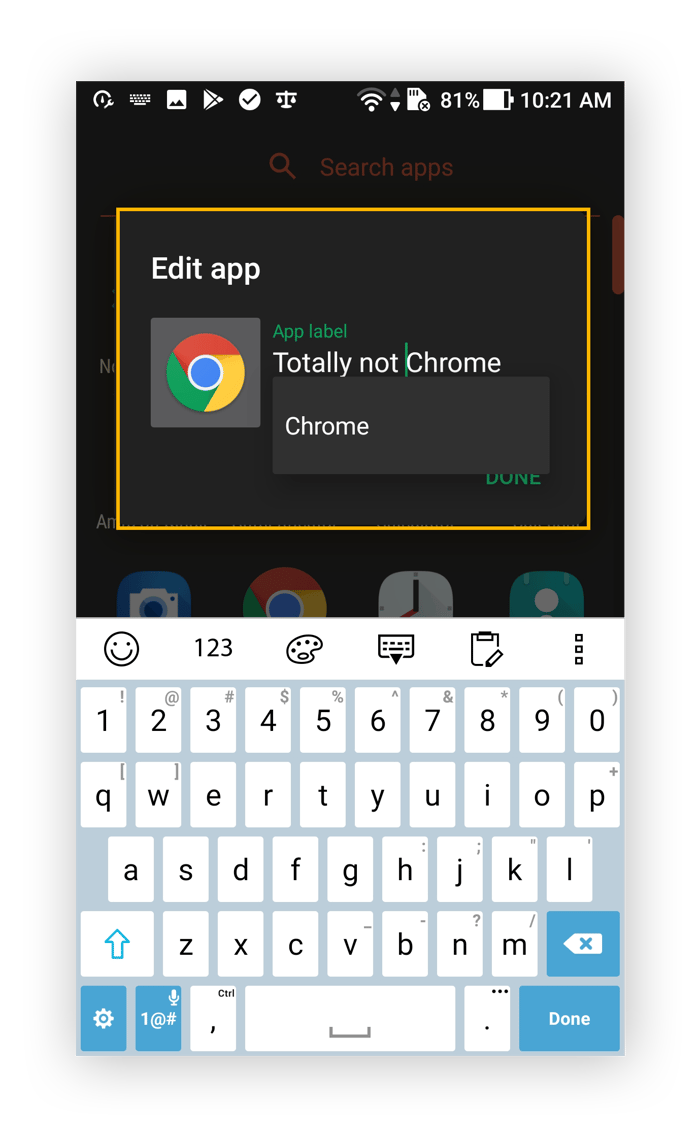The image, captured on an iPhone at 10:21 a.m. with 81% battery life and a strong connection, displays a busy screen filled with numerous icons at the top. The topmost section of the screen has a black header with a gold bar and the text "search apps." Below the gold bar, there is a gray box featuring a multicolored circular icon—resembling Google's logo with red, gold, green, and blue hues—next to the text "App label." This label is followed by the humorous text "totally not Chrome," with another smaller gray box containing the word "Chrome" above it. At the bottom of this smaller gray box, partially visible, is a button labeled "Done."

The central area of the screen shows four icon images arranged horizontally. Below these icons, the phone's keyboard is visible. The keyboard is predominantly white with traditional alphabet letters and numbers from 0 to 9. However, some keys, such as "return" and "done," are highlighted in blue. Above the keyboard, additional icons can be seen.